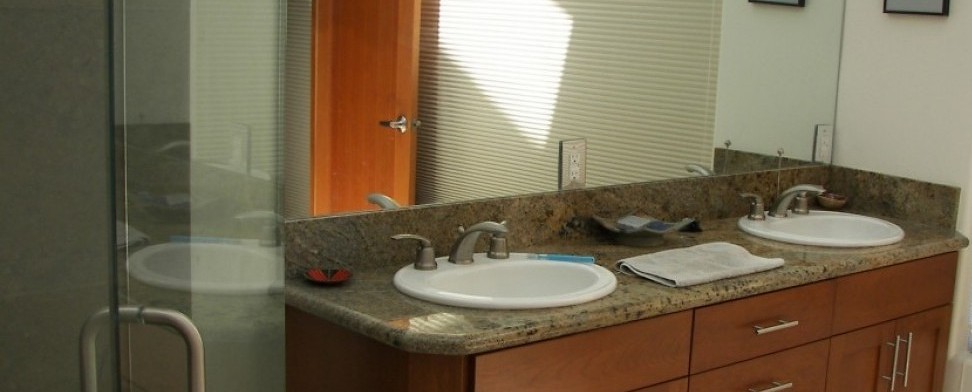This photograph captures a beautifully designed bathroom featuring a double sink vanity. Each of the two round, white sinks is set into a granite countertop characterized by its speckled pattern of gray, brown, and black. Below the countertop, brown cabinets provide storage space, adding warmth to the room's aesthetic. 

To the left side of the vanity, a walk-in shower is visible, enclosed by a glass door with a C-shaped metal handle. A large mirror spans the length of the vanity, interrupted only by an electrical outlet with a sleek mirror-finished plate, seamlessly blending into the reflective surface. 

A white towel is neatly placed between the two sinks, adding a touch of simplicity and cleanliness. On the far right side, a framed picture hangs on the wall, partially captured in the photograph, contributing to the room's tasteful decor.